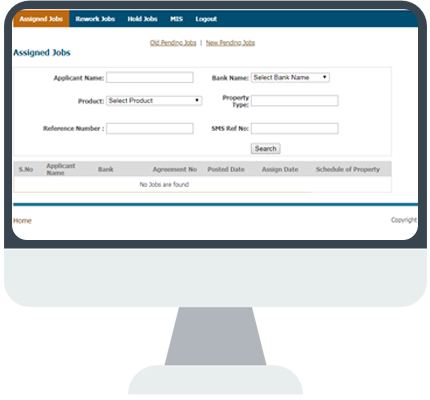The image depicts a computer monitor, resembling clipart typically used for illustrative purposes. On the left-hand corner of the screen, the header "Assigned Jobs" is barely legible due to blurred text. Adjacent to this header, a blue banner with indistinct words, possibly beginning with the letter "R" and ending with "Logout," is visible.

Beneath this header, centrally aligned text is separated by a line, with each line underscored. On the left-hand side, "Assigned Jobs" is prominently displayed in bold, blue font. A thin line divides this section from the next.

The next section begins with "Applicant Name," accompanied by a text box. To the right, a drop-down box next to an unreadable label, possibly "Bank Name," is present. Below, "Product" and "Select Product" along with their corresponding drop-down arrows are visible. The third line mentions "Product Type" with a text box, followed by "Reference Number" with another input box and an unreadable label with its corresponding box on the right. A "Search" button is positioned beneath these fields. The bottom of the screen features a gray banner containing additional, unspecified information.